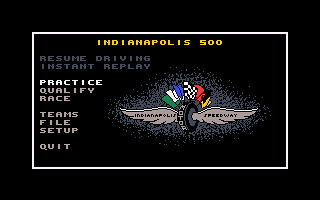This image is a screenshot from a video game, presented on a small screen. The background is a solid black, creating a stark contrast with the central rectangular gray box. At the top of this box, "Indianapolis 500" is prominently displayed in yellow text. Just below this, aligned to the left within the gray box, are several menu options listed in various colors: "Resume Driving" and "Instant Replay" rendered in light gray, then "Practice" in white. Continuing down the list, "Qualify," "Race," "Teams," "File," "Setup," and "Quit" are each written in gray. 

To the right side of the gray box, there's a logo featuring a tire centered between two angel-like wings, all shaded in varying tones of gray. Above this logo is an array of flags in multiple colors: green, white, blue, white and black checkered, red, black, and yellow, symbolizing different racing signals. The screenshot is somewhat small, which makes finer details, such as any possible text on the wings of the logo, difficult to discern.